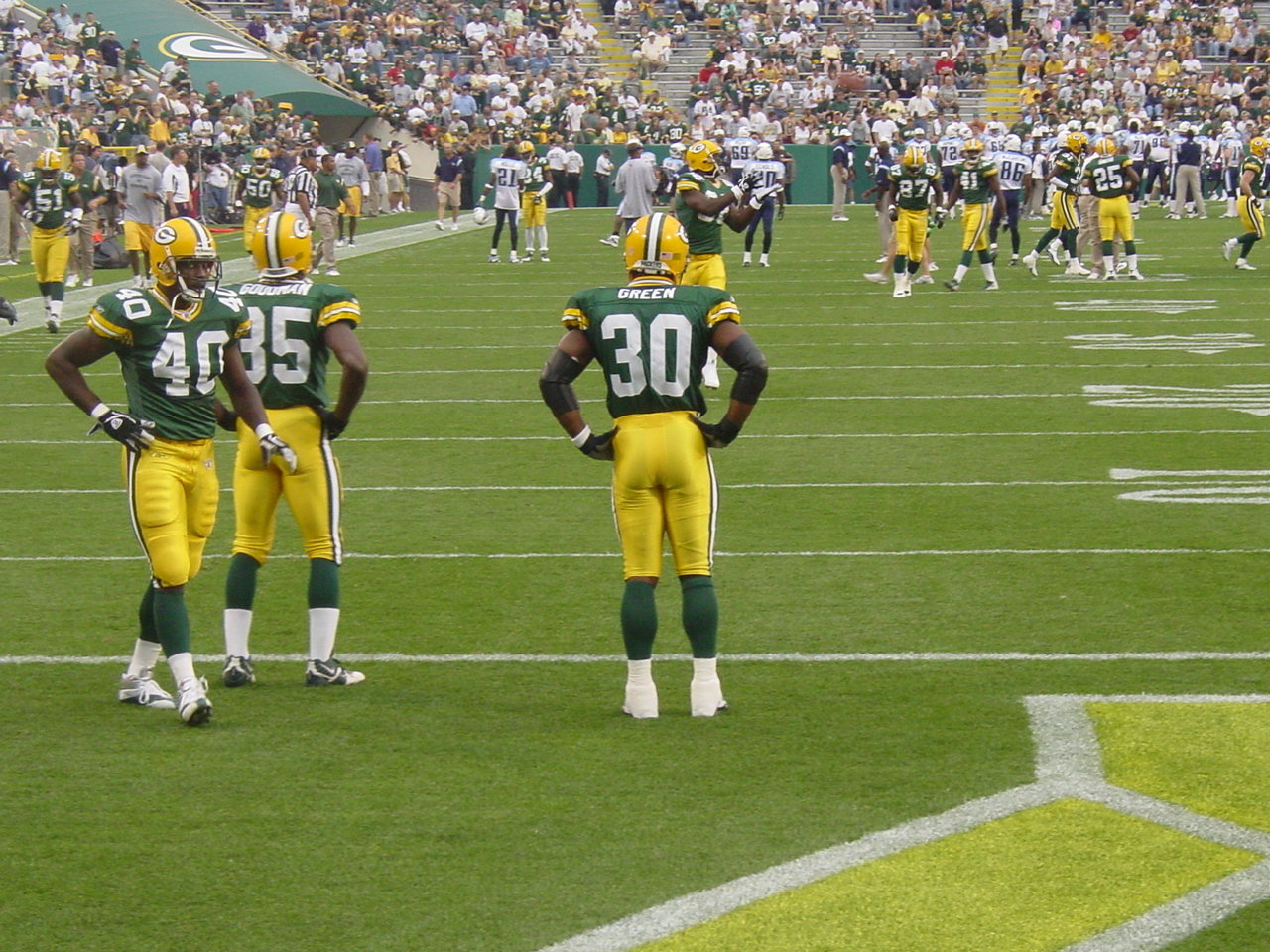This photograph captures an intense moment of an American football game between the Green Bay Packers and another team adorned in blue and white uniforms. The focus is on the foreground where three Green Bay Packers players stand out, especially player number 30, named Green, who is prominently positioned and wears green, navy, and white, with yellow spandex pants, high green socks, white shoes, and a green and yellow helmet. The field is marked with white lines and numbers such as 10, 20, 30, 40, and 50, leading to an end zone that features the Green Bay Packers' yellow symbol. 

In the background, a large, lively audience fills the stadium, predominantly dressed in Green Bay Packers colors, signifying a home game atmosphere. One Green Bay player appears poised with his hands up, ready to catch the ball, while another interaction shows a Packers player, number 34, shaking hands with an opponent. The image also captures the contrasting uniforms of the two teams, including Packers' players numbered 85, 87, and 25, with the opposing team’s players numbered 21, 34, 69, and so on. The action on the field is sharp and in focus, showcasing the dynamic motion and energy of the game, with vibrant green grass underfoot.